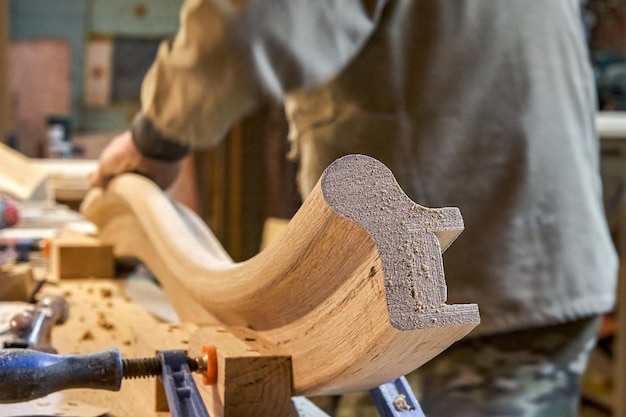In this color photograph of a woodworking shop, the focus is a large, long, wavy-shaped piece of light brown wood, partially rough on one side and smoothly sanded on the other. The wood is secured on a worktable using a black-handled tool with screws on both sides, preventing it from moving. Scattered around the table are numerous wood shavings and chips, indicative of ongoing craftsmanship. A person, whose head and face are not visible, is working on the wood. They are wearing a gray jacket with darker cuffs and camouflage green pants. Their left arm gently rests on the wood while they stand with their back towards the camera. In the blurred background, a brown patterned wall is partially visible, adding texture to the scene. The workspace is cluttered with various tools and equipment left on the table, emphasizing the busy, industrious environment of the shop.